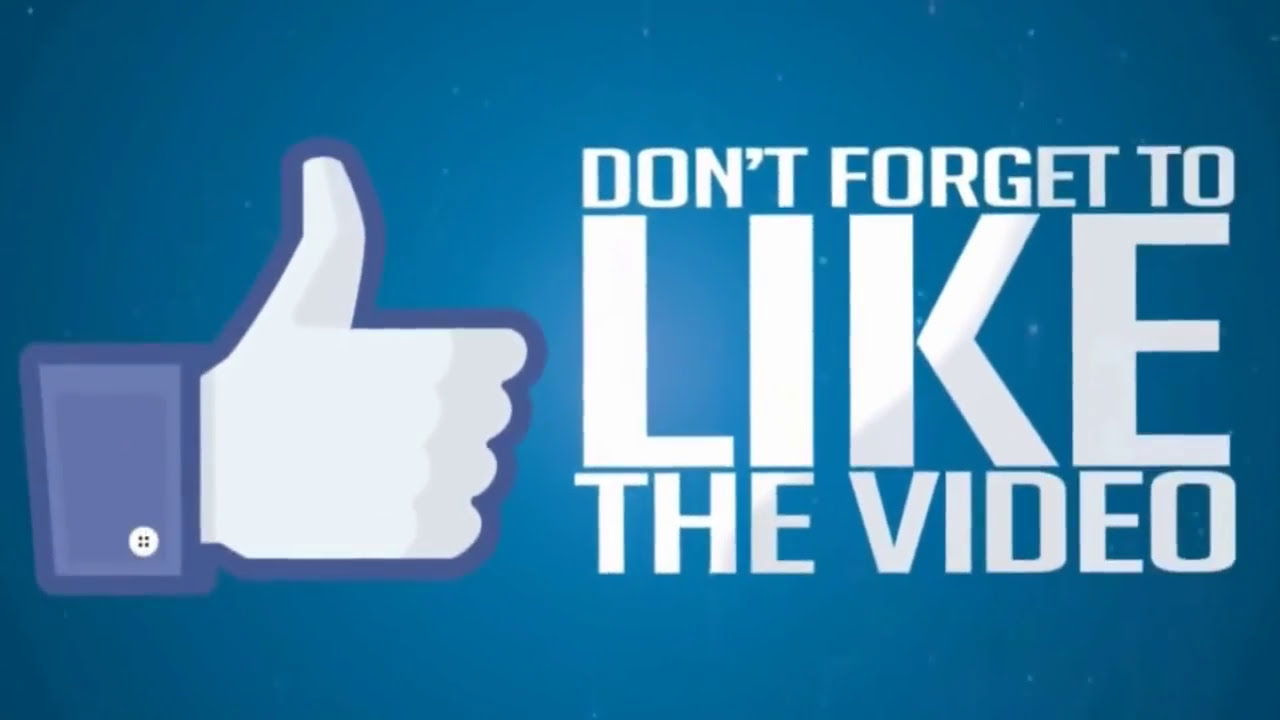The close-up image resembles a final frame you might encounter after watching a YouTube video. It has a blue background that fades from a lighter blue in the center to a darker blue at the corners, with tiny white specks scattered throughout, reminiscent of a sky. On the left side of the image is a large white hand giving a thumbs up, adorned with a blue cuff and white button on the wrist. To the right of the hand, in all-capitalized white text with a subtle blue aura, the text reads "DON'T FORGET TO" at the top, "LIKE" in much larger font beneath it, and "THE VIDEO" in medium-sized font below "LIKE." The overall message of the sign is a prompt for viewers to "Don't forget to like the video."